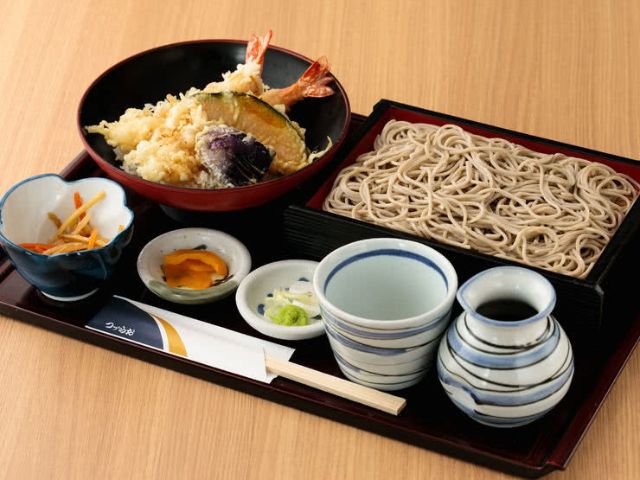The image is a detailed color photograph showcasing a variety of food items artfully arranged on a light brown wood veneer table. The food is presented on a rectangular, black lacquer tray. In the upper left corner of the tray, there is a red bowl with a black interior containing fried shrimp tempura along with some fried vegetables, including eggplant and sweet potato.

Adjacent to this, a rectangular dish holds a serving of brown soba noodles. Nearby, there is a blue and white cauldron-shaped vase, and a matching mug with the same color scheme is situated on the bottom left. 

The foreground features five circular dishes with different items. One dish contains pickled vegetables, another holds wasabi, and the next has slices of ginger and possibly pickled carrots or onions. There is also a bowl with sweet potato fries and a small white bowl with guacamole. Another small white bowl holds what appears to be peaches. The tray additionally includes a black and brown bowl filled with rice and a portion of battered fish.

To the right, there is a square plate with thin lo mein-style noodles, and a round cup likely intended for tea or water is also present. Completing the presentation, a pair of wooden chopsticks rests at the bottom of the tray, contributing to the meticulous and aesthetic arrangement of the image.